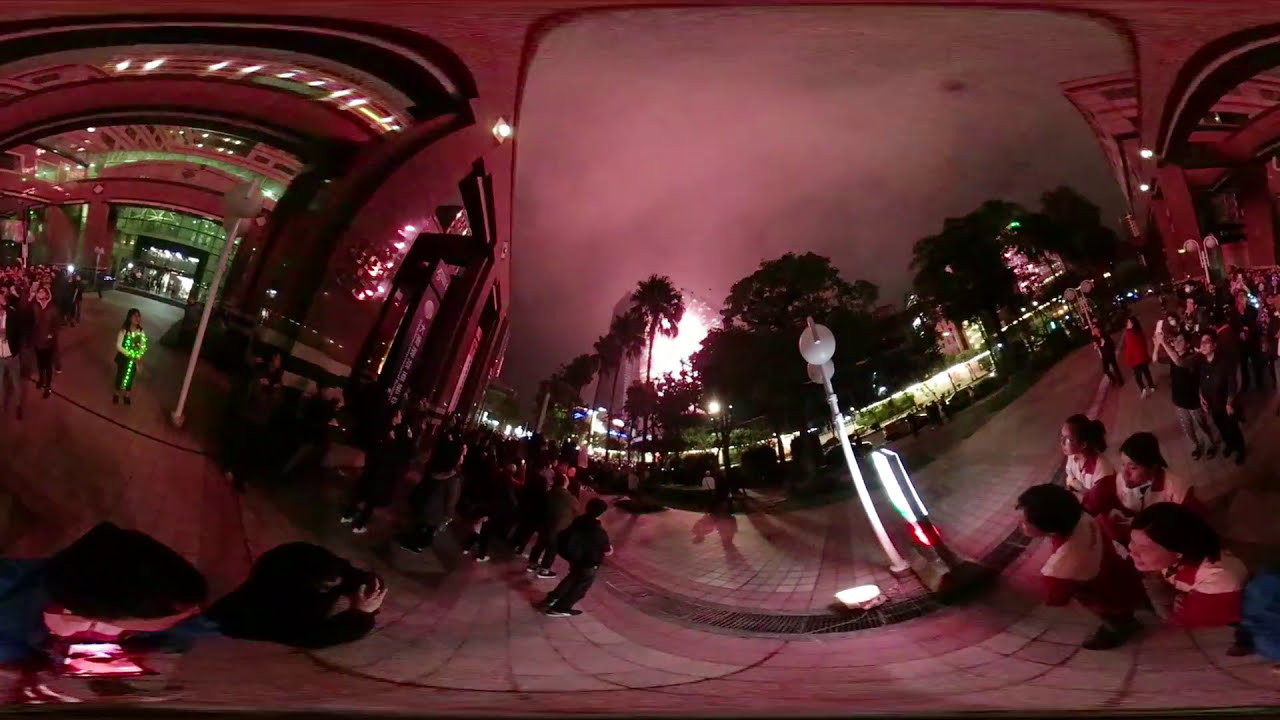This is a panoramic fisheye lens photograph taken in a bustling downtown area at night, characterized by an unusual purplish-red hue, possibly due to a filter or the type of lighting. The sky above is overcast, appearing almost gray-black, amplifying the nocturnal atmosphere. Prominently to the left side of the image is a large mall-like building with a vast glass entrance framed in dark-colored material. Standing under an archway leading up to this entrance, a woman is adorned with vibrant green string lights, resembling a festive ornament.

The pathway is crowded with multiple people walking, some of whom have their phones pointed upwards towards the center of the photograph, where a large light is emanating from the ground. Towards the lower right corner, several young individuals dressed in sports uniforms are gathered, possibly fans near a stadium entrance. They stand on a stone sidewalk made of square bricks and are in front of a lit sign. The background reveals a line of trees and a distant cityscape emerging through the night.

Palm trees occupy the central area of the image, adding to the diverse flora. Notably, there are Chinese or Japanese characters visible on one of the buildings towards the left, suggesting that this scene is set in an Asian metropolis. The overall scene melds outdoors with an expansive lobby space, creating an intriguing visual effect that captures the dynamic essence of a lively urban night.